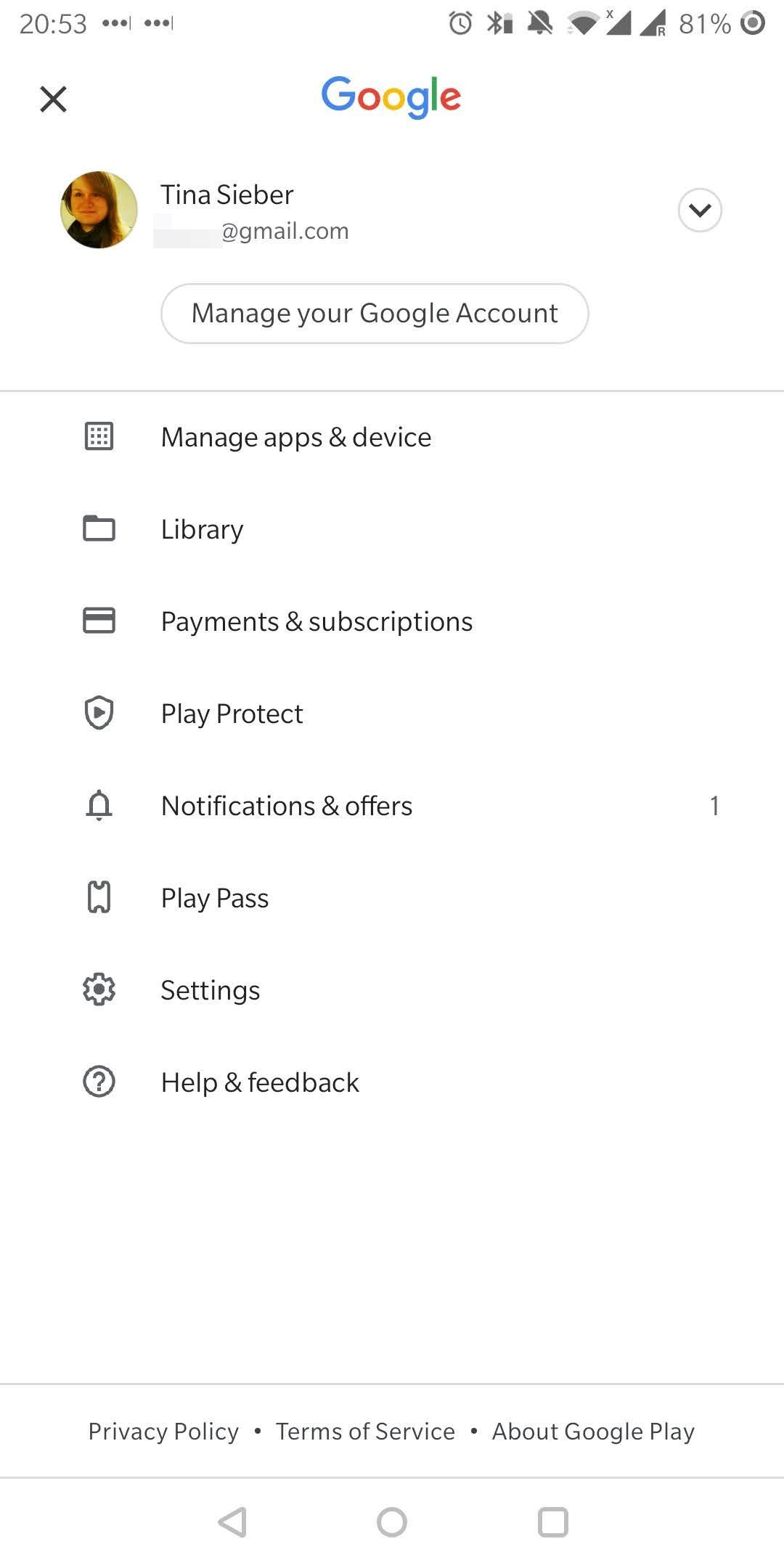The image depicts a Google account management screen for illustrative purposes, featuring the account of Tina Sieber (tina.sieber@gmail.com). The interface is clearly identifiable as a Google product, highlighted by the prominent Google logo at the top. The current time displayed on the screen is 20:53.

Below the time indicator, there is a list of options available for managing the Google account, each accompanied by a distinctive icon on the left-hand side. The options include:

1. **Manage apps and devices** - Represented by a square icon with dots.
2. **Library** - Symbolized by a folder icon.
3. **Payments and subscriptions** - Marked with a credit card icon.
4. **Play Protect** - Shown with a shield badge icon featuring a play button at the center.
5. **Notifications and offers** - Indicated by a bell icon.
6. **Play Pass** - Depicted with a unique icon resembling an upside-down W on top and a back-to-front W at the bottom, styled within a rectangle.
7. **Settings** - Represented by a cogwheel icon.
8. **Help and feedback** - Identified by a circle icon containing a question mark.

This structured and detailed visual provides an organized overview of various account management functionalities available to the user.